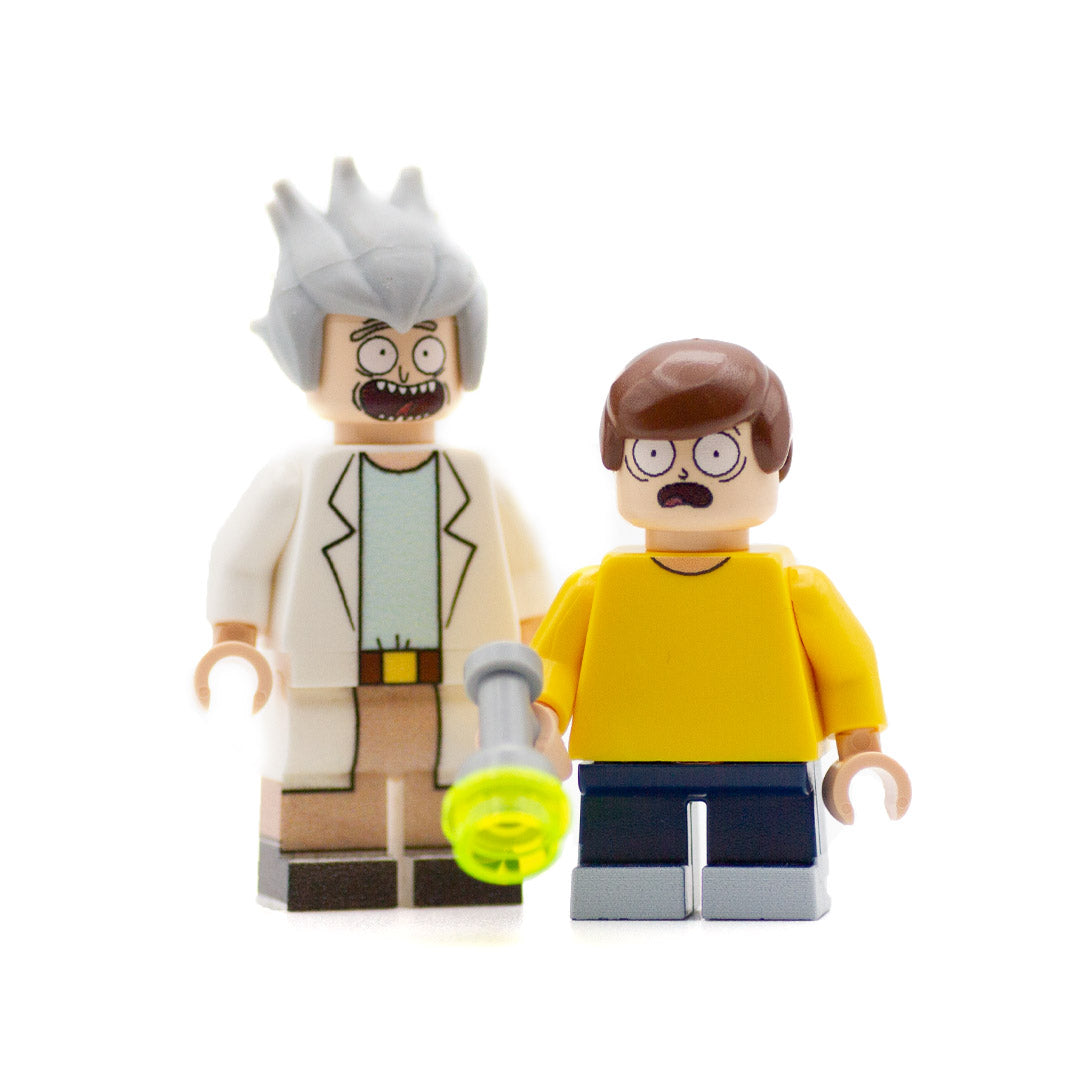This image is an up-close, color photograph of two customized Lego figurines depicting Rick and Morty from the animated series "Rick and Morty." On the left stands Rick, characterized by his spiky gray hair and an excitable expression with his mouth open, showing teeth. He is outfitted in a white lab coat over a light blue t-shirt, tan pants, a tan belt with a brass buckle, and black shoes. Rick holds a neon green-tipped portal gun in his left hand. To his right is Morty, identifiable by his short brown combed-over hair and his worried expression, his mouth noticeably downturned. Morty is dressed in a yellow short-sleeved shirt and blue jeans, and he clutches a Lego blaster gun. Both figures feature the iconic rounded Lego hands. The background of the image is transparent, free from any lines or additional elements, emphasizing the detailed and vivid portrayal of these beloved cartoon characters.